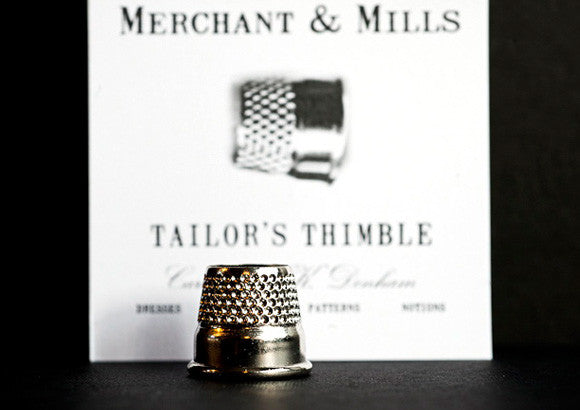The image depicts a small silver thimble, positioned on its side with the open part resting on a glossy black surface. The thimble is highly textured with uniformly spaced dimples covering its top half, and it has a solid lip at the bottom. The background is entirely black, except for a vertically oriented white card that stretches to the top of the frame. The card displays the text "Merchant and Mills" in black font at the top, followed by an illustration of the thimble on its side, and underneath it reads "Taylor's Thimble." Any additional text on the card is blurred and indistinguishable. The clarity and shininess of the thimble contrast sharply with the blurred details on the card and the deep black background, making the thimble the focal point of the image.